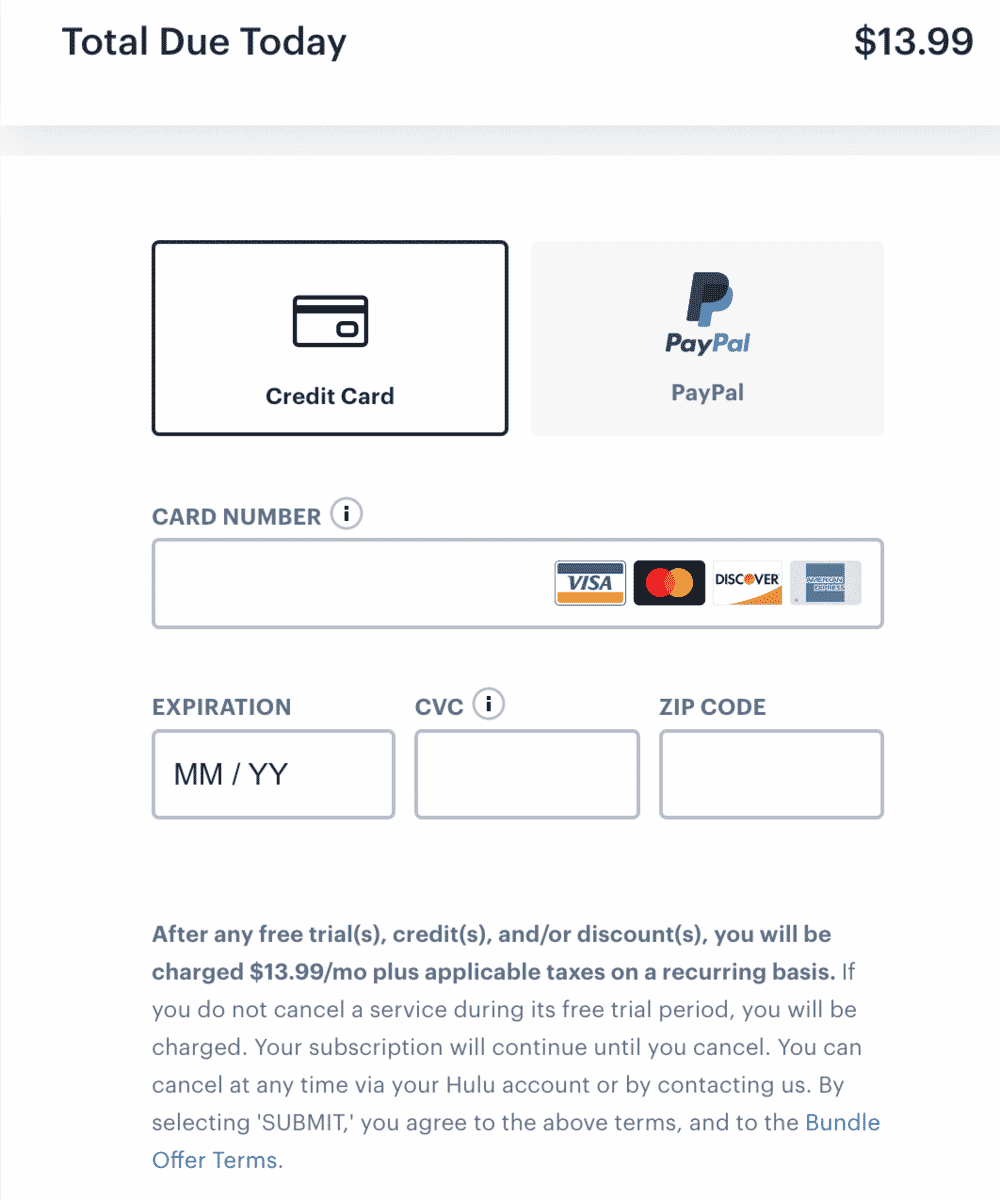This image depicts an invoice for a Hulu subscription. At the top, the total amount due today is displayed prominently: $13.99. Directly below this is a gray bar, beneath which the word "Credit Card" along with a credit card icon is shown on the left. To the right, there is a PayPal icon. The credit card option on the left is the one highlighted.

Below this section, the label "CARD NUMBER" appears in all capital letters, with an information icon (a circled "i") next to it, indicating that additional information is available. There is a field provided for entering the card number with options for Visa, MasterCard, Discover, or American Express.

Following this, three fields for payment details are displayed: "EXPIRATION" (indicating MM/YY for the month and year), "CVC" (with another information icon), and "ZIP CODE," all in capital letters.

Further down, a bolded statement clarifies the billing terms: "After any free trials, credits, and/or discounts, you will be charged $13.99 a month, plus applicable taxes on a recurring basis. If you do not cancel the service during the free trial period, you will be charged. Your subscription will continue until you cancel. You can cancel at any time via your Hulu account or by contacting us." 

It concludes with a prompt: "By selecting SUBMIT (in all capital letters), you agree to the above terms and to the bundle offer terms."

This form appears to be set up for the payment of a Hulu subscription at a rate of $13.99 per month plus applicable taxes, following a free trial period. The free trial might have ended, requiring the user to now pay for the service to continue their subscription.